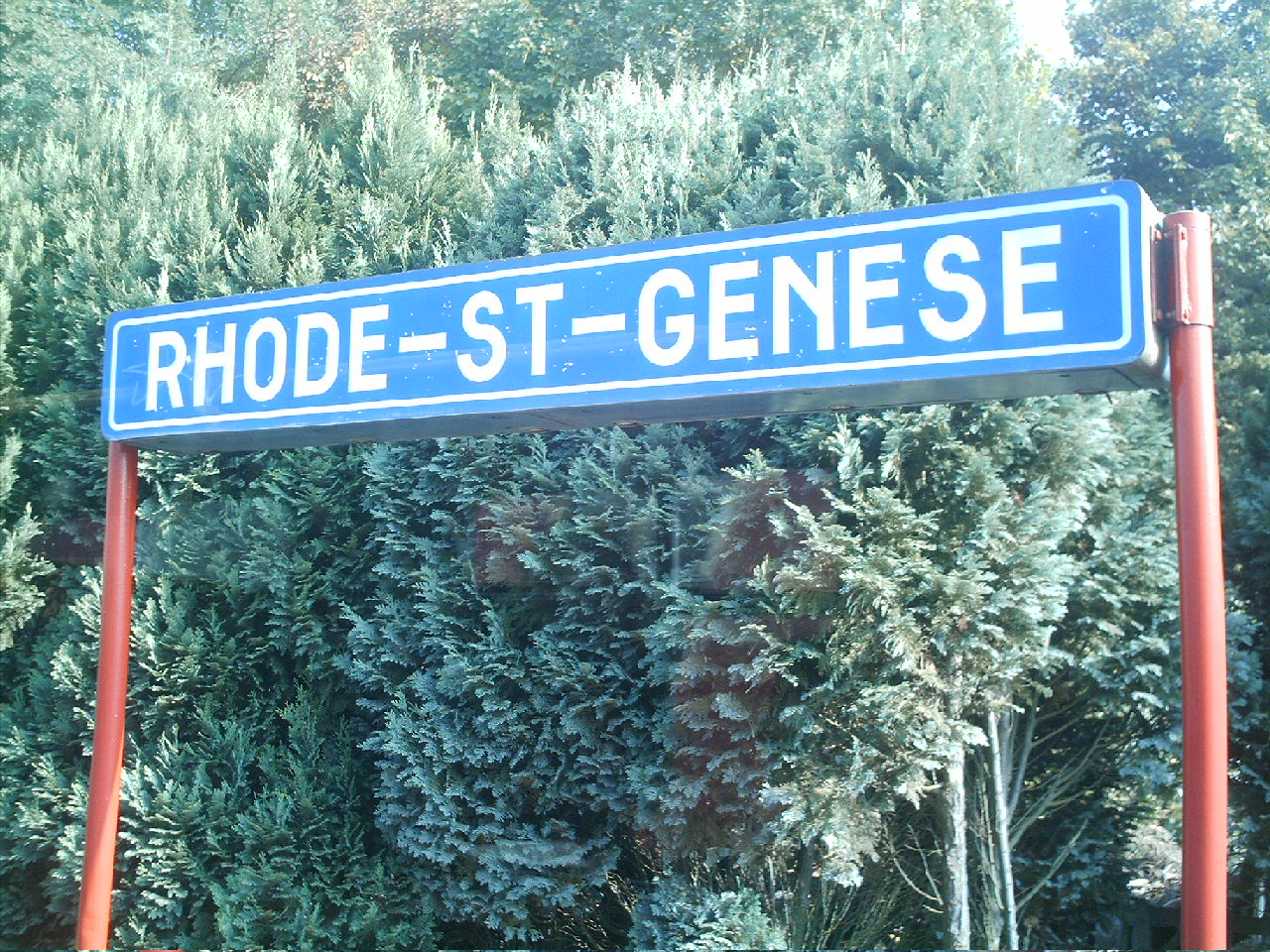This is a landscape-oriented photograph featuring a prominent advertisement sign for a facility. The sign itself is a solid blue, mounted on two sturdy poles that are either red or a reddish-brown hue. The sign extends horizontally, with a white rounded rectangle centrally positioned on the blue background, which is accented by a white outline. Within this rectangle, bold sans-serif text reads "ROAD-ST-GENESE," the name of the place.

The backdrop is predominantly composed of a dense array of trees, giving the impression of a heavily wooded area. This photograph was taken during daylight hours, as evidenced by the natural lighting filtering through the scene. The image seems to be captured from within a vehicle, discernible by the faint reflections and glares on the window, or possibly there are spider webs or other natural structures visible among the trees, contributing to the lighting patterns observed.